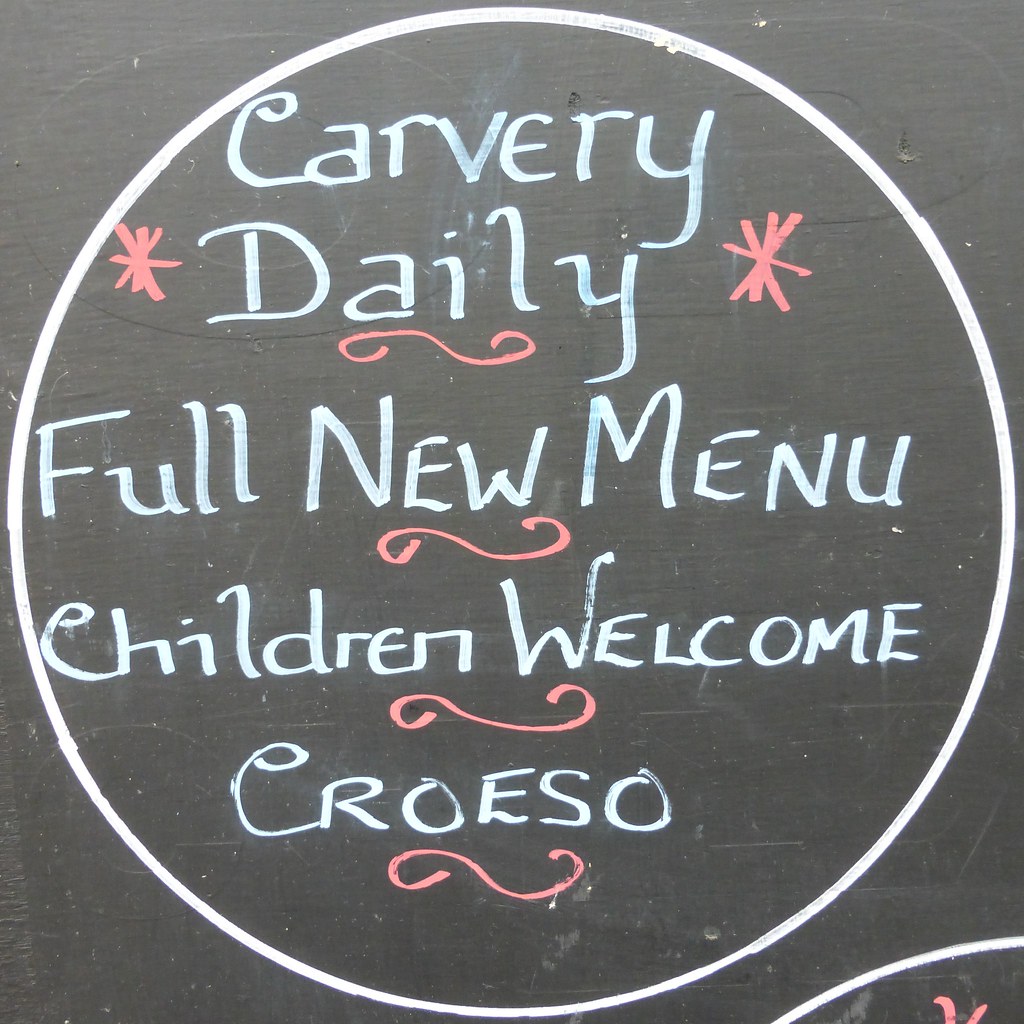This image appears to be a blackboard advertisement typically seen outside a restaurant, showcasing a chalkboard surface with a dark gray, almost black, textured background. In the center is a large white circle framing the handwritten text, which is presented in a pale blue or white color. The text reads: "Carvery Daily" on the first line, embellished with two pink asterisks adjacent to "Daily." Below that, "Full New Menu" is featured on the second line, followed by "Children Welcome" on the third line. Each of these phrases is underscored by a dark pink squiggly line. At the bottom, "Croeso" (spelled C-R-O-E-S-O) appears, also underlined with a pink squiggly line. This detailed and decorated presentation likely aims to draw attention to the restaurant’s offerings and welcoming atmosphere. In the bottom right corner of the image, part of another circle and star is visible, suggesting additional elements of the menu or advertisement not fully captured in this image.